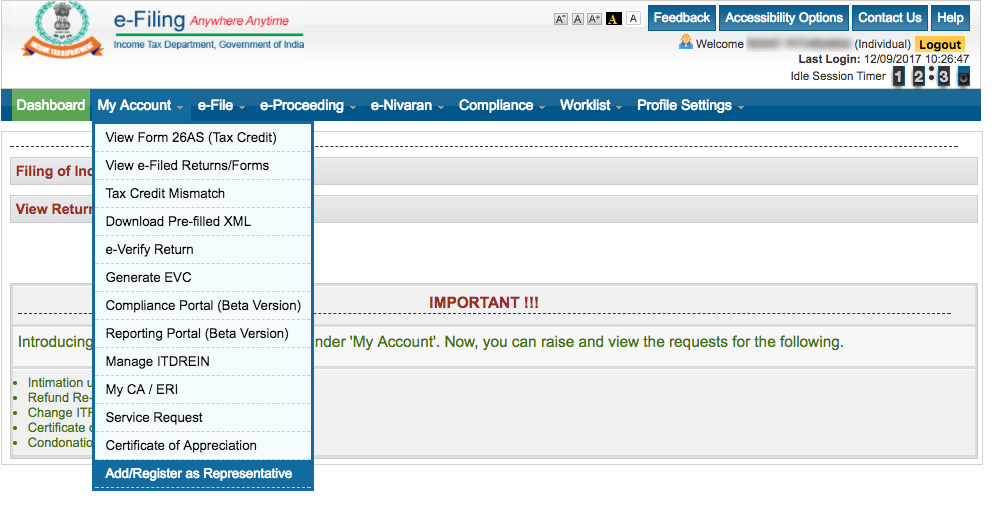Screenshot of the Indian Income Tax eFiling Website

This screenshot captures the homepage of the Income Tax Department eFiling website for India. At the top-left corner, the header features the label "eFiling" in blue, accompanied by the phrase "Anywhere Anytime" in red. Just below it, the text "Income Tax Department, Government of India" is displayed. An emblem is also present in the upper left corner, consisting of a blue circle with an indistinct grey object resembling a tower, and an orange ribbon beneath it.

On the right side of the navigation menu, there are rectangular blue buttons with white text labeled "Feedback," "Accessibility Options," "Contact Us," and "Help." The background color of the main navigational menu is blue, with white font used for the menu items. Notably, the "Dashboard" item is highlighted in green, while the rest of the menu items, including "My Account," "eFile," "eProceeding," "eNiravan," "Compliance," "Worklist," and "Profile Setting," are in blue.

A dropdown menu has been selected under "My Account," revealing a detailed list of options. The first item listed is "View Form 26AS" with "Tax Credit" indicated in parentheses. The list appears to be extensive, continuing down the page.